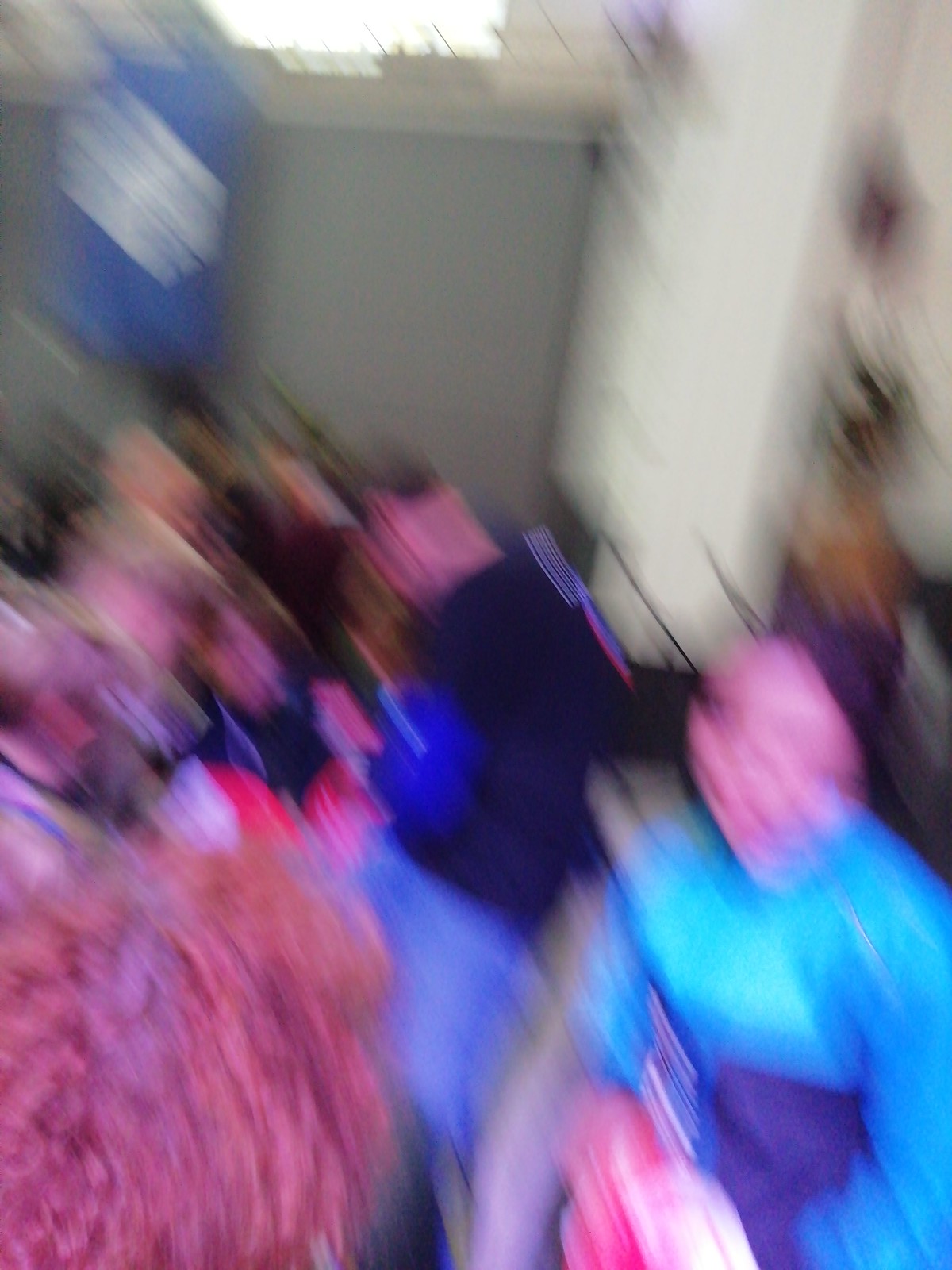The image is significantly blurred, suggesting motion while the picture was taken. It appears to have been captured indoors, as indicated by the architectural features visible in the background. Towards the back, there is a vaguely discernible white post and a variation in wall color, which includes a window positioned higher up. Near this window, a bluish object hangs down, adding a bit of color contrast.

In the main area of the image, there seem to be at least five individuals, possibly more, though the blur makes exact numbers difficult to distinguish. On the bottom right corner, one can see a person wearing a blue shirt. Nearby, another individual stands out in a black shirt. The rest of the image shows a group of people who are either standing or seated, aligned in a row, though their details are obscured due to the blurriness.